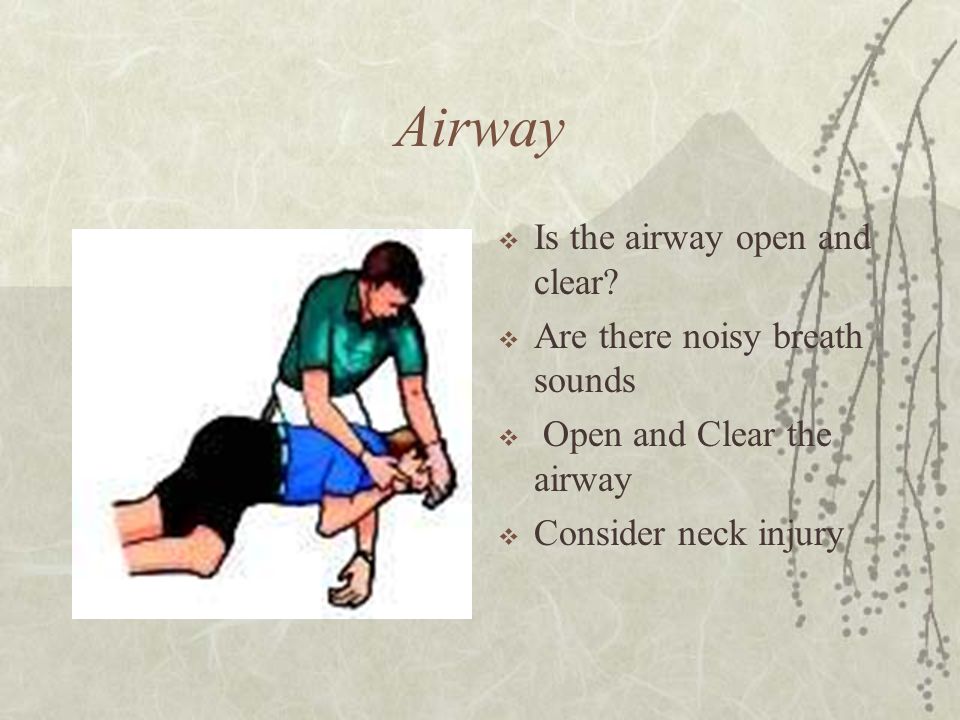In the image, a man wearing a short-sleeved green shirt and white pants appears to be performing CPR or administering care to a woman who is sprawled out on her side. The woman is dressed in a short-sleeved blue shirt and black shorts. Both individuals have light peachy skin tones. The man has black hair, while the woman has brown hair, and they are each wearing wrist accessories. At the top of the image, the word "airway" is displayed in italicized Times New Roman font with four bullet points beneath it. The bullet points read: "Is the airway open and clear?" "Are there noisy breath sounds?" "Open and clear the airway." and "Consider neck injury." The background is beige, featuring a dull gray mountain range and branches studded with berries drooping from the top right corner.